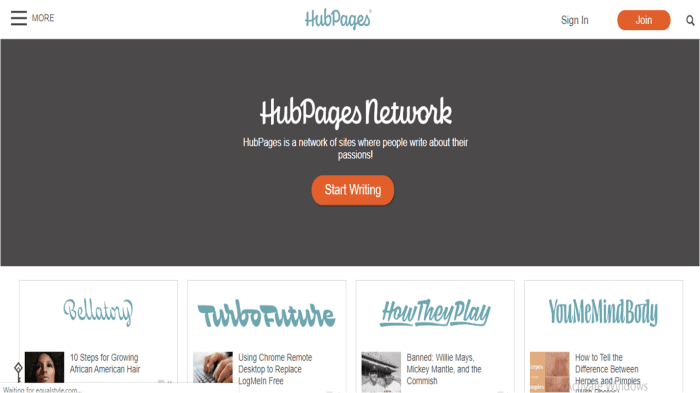The landing page for the HubPages Network features a prominently dark charcoal black rectangle centered on the page, with "HubPages Network" in elegant white script positioned centrally. Below this, white descriptive text reads, "HubPages is a network of sites where people write about their passions." Directly beneath the description, an inviting orange action button with white text, "Start Writing," and rounded corners is displayed.

At the very top of the page, a standard header bar spans across, beginning on the left with three horizontal lines and the word "More" in all capital letters. Centered in the header is the blue HubPages script font trademark logo. On the right side, there is a "Sign In" button, which is a white button with black text, and a "Join" button, an orange button with white text. Located in the upper right corner is a search magnifying glass icon.

The bottom section of the page is divided into four distinct panels, each delineated by thin gray square boundaries and featuring different panel titles in a script futuristic font. The first panel is titled "Bellatory," displaying a picture of a woman with the caption, "10 Steps for Growing African American Hair." The second panel, "TurboFuture," features a photo of hands on a keyboard with the text, "Using Chrome Remote Desktop to Replace Log Me In Free." The third panel, "How They Play," showcases a playful underlined script with an old photo of two baseball players in a stadium, captioned "Bonds, Willie Mays, Mickey Mantle, and The Commish." The final panel, "You, Me, Mind, Body," features closely spaced words and a picture resembling the light brown or orange cover of a book, with partial text, "How to Tell the Difference Between Herpes and Pimples."

Each element on the page is thoughtfully positioned, offering a clear and engaging user interface for visitors interested in exploring or contributing to the HubPages Network.